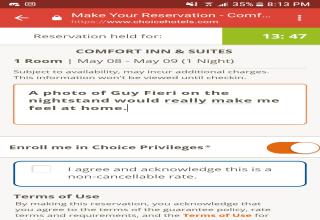This is a screenshot from a mobile phone displaying a reservation confirmation page for Comfort Inn & Suites. The top header is red and prominently displays the title: "Make Your Reservations Comfortable." Below the header, there is a section titled "Reservation Held For," which features a green box on the left side displaying the military time "1347," equivalent to 1:47 PM. 

The reservation details indicate a stay at Comfort Inn & Suites, booking one room for the night of May 8th through May 9th. A white text box features the phrase: "A photo of Guy Fieri on the nightstand would really make me feel at home," and a cursor is visible at the end of the sentence. 

The next section offers an option to "Enroll me in Choice Privileges," highlighted by an asterisk and toggled on with a yellow and orange switch. Below this, a blue-outlined checkbox states, "I agree and acknowledge this is a non-cancellable rate."

At the very bottom, the "Terms of Use" section is written in red text and spans about four lines.